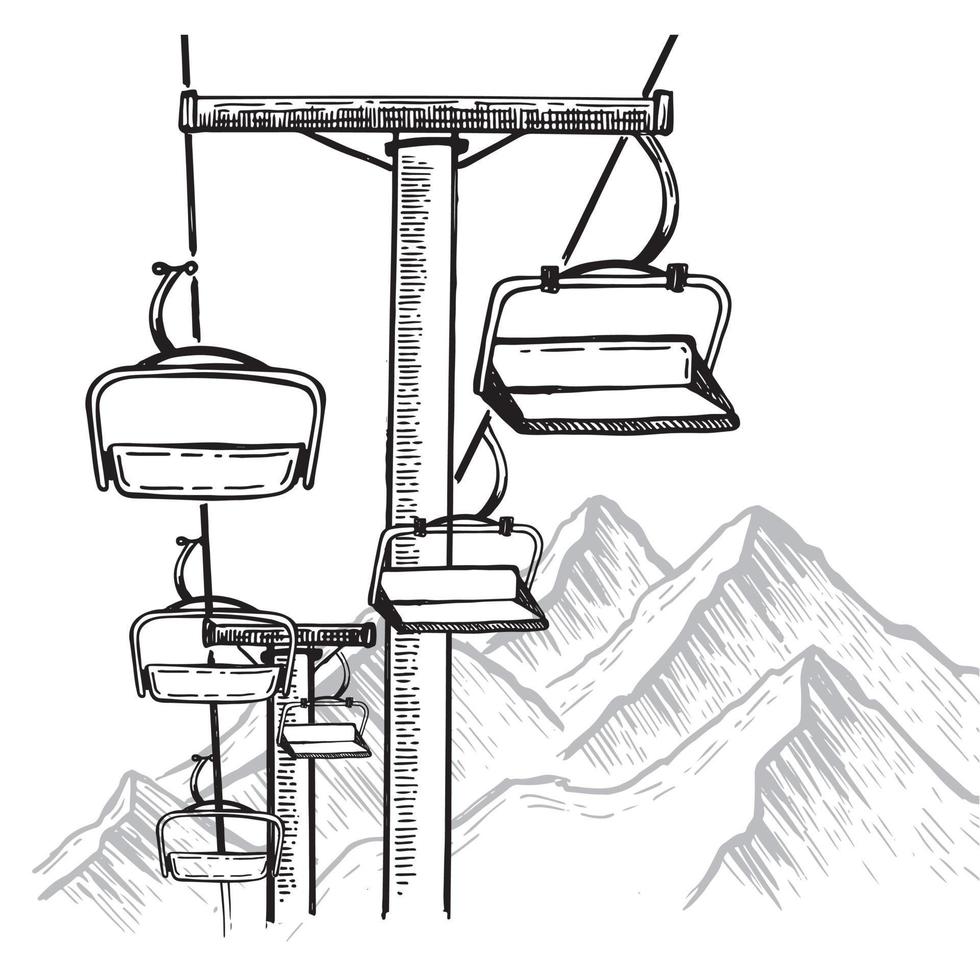This monochromatic line art illustration depicts a ski lift, where six empty chairs are visible—three ascending and three descending the mountainside. The ski lift's components, including the haul rope, carriers, and supporting towers with textural cross-hatching, are rendered in bold black lines, giving them prominence against the stark white background. The backdrop features a range of light gray mountains with subtle cross-hatching and dashes that evoke a bare-bones texture, creating a sense of distance and simplicity. The mountain peaks are skewed slightly to the right and reach just under halfway up the image’s height. This detailed yet minimalist representation, with no people or text, highlights the sharp and clean contrast between the ski lift's intricate mechanics and the serene, subdued mountainous landscape.